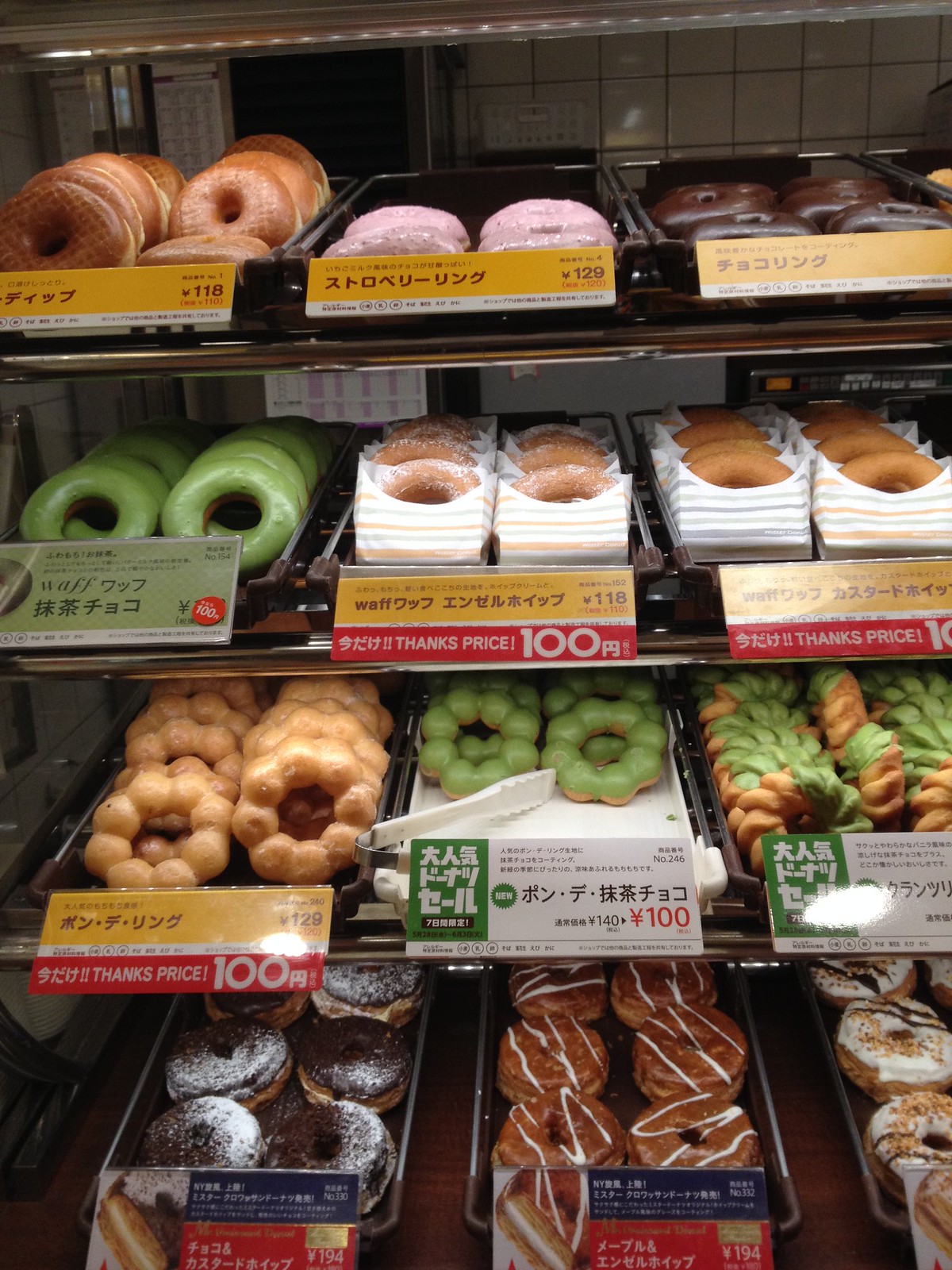This detailed photograph captures the enticing view through the front glass of a bakery's donut display cabinet, showcasing four brown shelves, each with three dark-colored trays holding approximately eight to twelve donuts. The trays have labels in front of them featuring writing in red, white, and black, with the top part of the label being yellow and the bottom part white on the first row, and green, white, red, and yellow with white lettering on the second row. The labels seem to include both English and Asian characters, possibly Japanese or Chinese, providing descriptions and pricing information.

The wide variety of donuts displayed include honey dip, chocolate glaze, and green frosting options. Notably, there's a French cruller style, a Boston cream style donut on the bottom left, and crumbly style donuts on the far right. Some donuts are adorned with white icing and black swirls, while others are powdered with sugar, plain, or have pink icing, especially visible at the top center. Among the assortment on the third shelf down to the left, there is a unique donut configuration made of small balls of dough joined together with a hollow center, resembling flower petals.

The overall display is inviting, with each shelf presenting a colorful and diverse array of flavors and styles that are sure to tantalize the taste buds of anyone peering into this bakery cabinet.